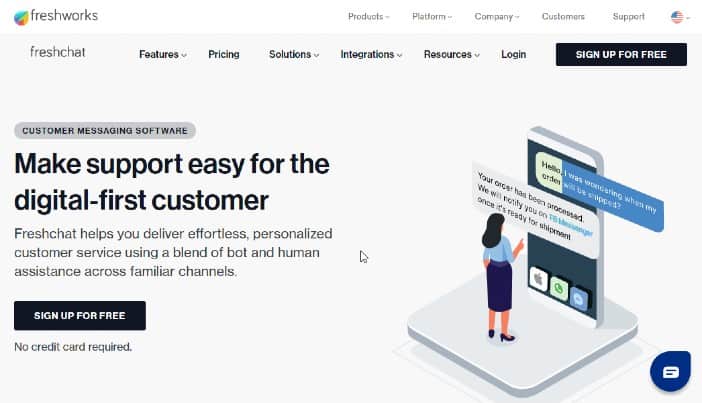In the Siemens example, the image depicts the landing page of a website. At the top, there is a logo with blue and yellow rounded edges, labeled "Freshworks." To the right of the logo, there are clickable sections for "Products," "Platform," "Company," "Customers," and "Support." Below the "Freshworks" logo, the text "Fresh Chat" is prominently displayed. Further to the right, additional options are visible, including "Features," "Pricing," "Solutions," "Integrations," "Resources," and "Login." A black box with white text appears below these menu items, offering a "Sign up for free" option.

On the right side of the page, there is an animated illustration of a woman dressed in a blue shirt and blue skirt with long dark hair. She is interacting with a giant smartphone, which displays a chat interface. The chat messages read: "Hi, hello, I was wondering when my order will be shipped?" and a response saying, "Your order has been processed. We will notify you [text cut off] once it’s ready to be shipped." The setup suggests this is a customer service platform focused on handling shipping inquiries.